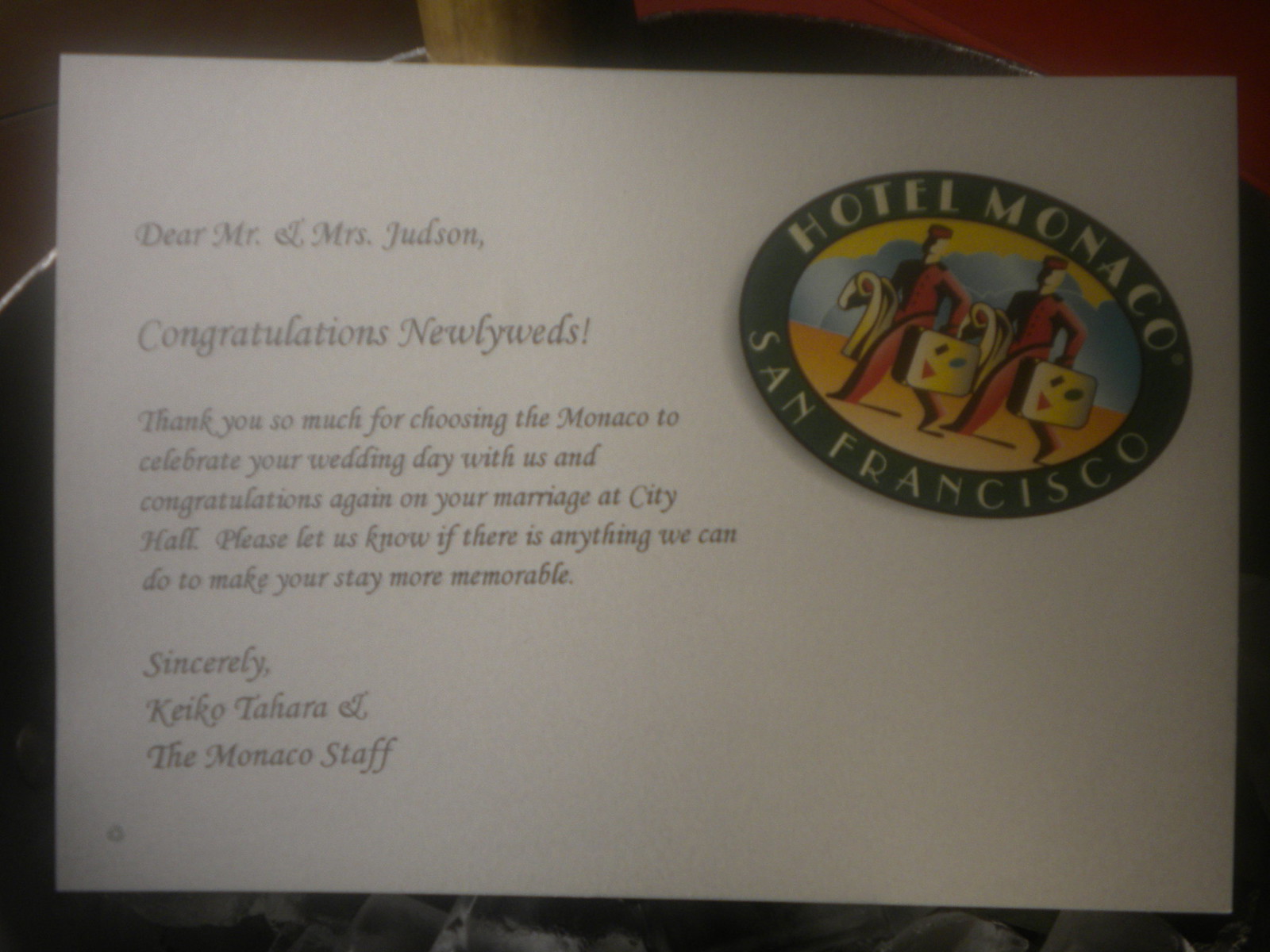The image depicts a somewhat dark and blurry piece of paper, bearing multiple lines of black text. Situated in the top right corner of the paper is a cartoon-like graphic within a dark green oval border, featuring two people in red uniforms holding a suitcase and coat, denoted as the logo for Hotel Monaco, San Francisco. The text on the paper reads: 

"Dear Mr. and Mrs. Judson, 

Congratulations, newlyweds! Thank you so much for choosing the Monaco to celebrate your wedding day with us, and congratulations again on your marriage at City Hall. Please let us know if there is anything we can do to make your stay more memorable. 

Sincerely, 

Keiko Tahara, the Monaco staff."

The handwriting appears fancy with additional decorative designs on the letters. The letter spans across the left side of the paper, providing a warm and personal message from the hotel staff to the newlywed couple. The overall aesthetic gives the impression of a thoughtful and formal congratulatory note from the hotel.